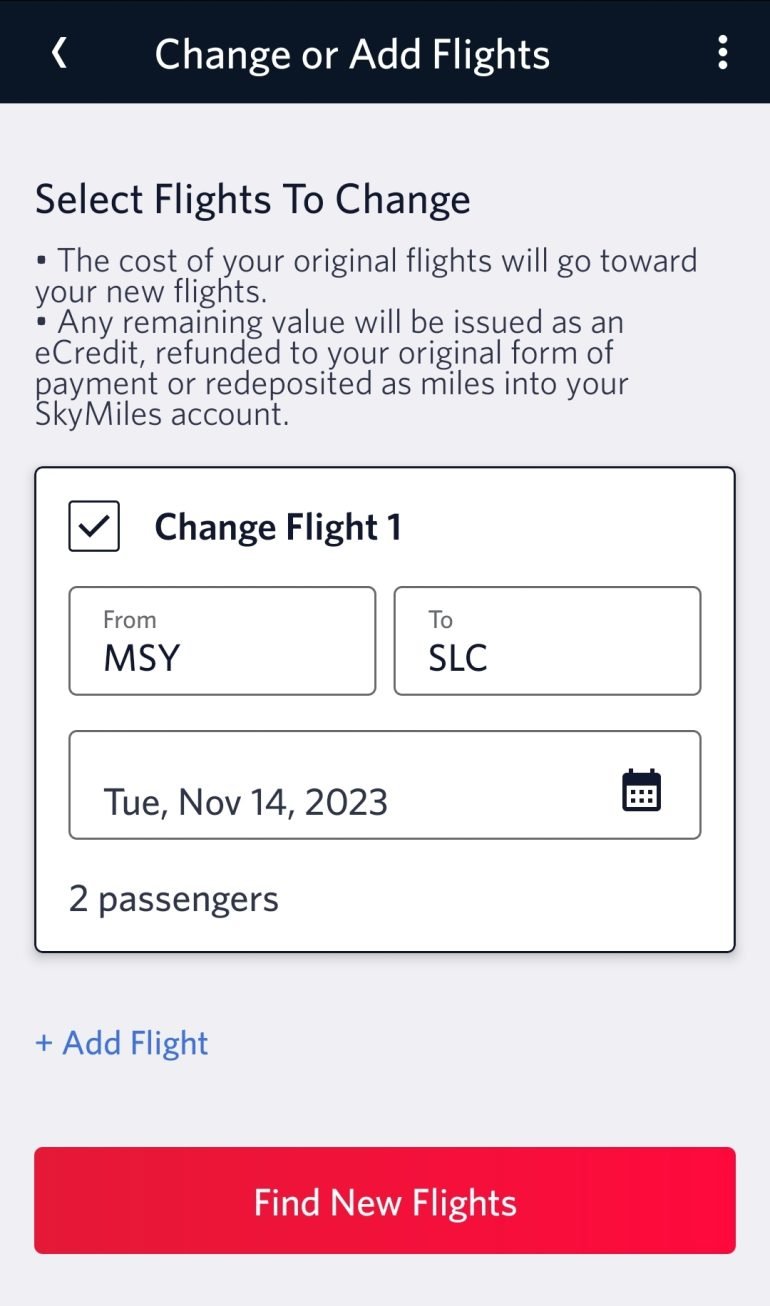The image is a detailed interface for modifying flight reservations. The lower section of the interface is black, transitioning to the upper section which features a white area ending in an arrow pointing to the left. In this white section, the text reads "Change or Add Flights" with three adjacent white circles serving as decorative or functional elements. Above this, the background shifts to a light gray color.

Displayed prominently on the gray background in dark gray text is the instruction "Select Flights to Change." Below this are two bullet points outlined in black. The first bullet point explains, "The cost of your original flights will go towards your new flights. Any remaining value will be issued as an eCredit, refunded to your original form of payment, or redeposited as miles into your SkyMiles account."

Next to this bullet point is a white box with a black outline, containing a black checkmark, indicating a selection status. The text "Change Flight 1" appears in black next to this checkbox.

Underneath, the first bullet point contains two rectangles: the first one in gray reads "ROM," and in black, it states "MSY." The second rectangle, also in gray, displays "To." Below this in black, it lists "SLC."

Further down, another white rectangle with a black border contains the text "TUE," followed by "Tuesday, Nov 14, 2023," also in black. This section is accompanied by a small calendar symbol in native blue and white.

Beneath this, the text "2 passengers" appears in black. Following a gray space, there is a blue text "+ Add Flight." Finally, a red rectangle at the bottom of the interface reads "Find New Flights" in white text with each word capitalized.